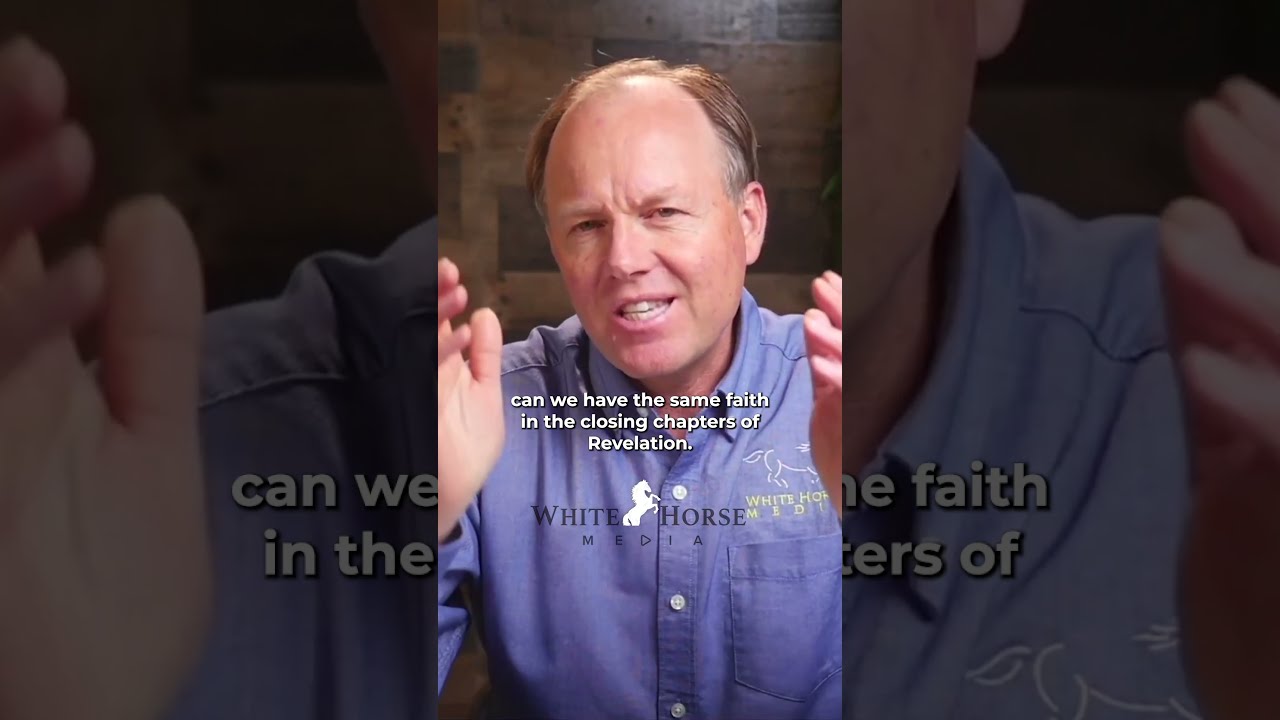The image is a composite featuring a central photograph of a man set against slightly shadowed sections on the left and right. The central figure, who has a solemn expression with his mouth slightly open and his eyes squinted, appears to be speaking. He has a receding hairline, with brown hair that is short at the sides. The man is wearing a blue button-up shirt with white buttons, emblazoned with "White Horse Media" and a symbol of a white horse. He holds both hands up on either side of some text that reads, "Can we have the same faith in the closing chapters of Revelation?" In the background, a wooden wall with varying tones of beige and brown serves as a backdrop, giving an impression of either slatted or pallet-style construction. The image also includes zoomed-in sections showing the man's right side of the face and hands, as well as a close-up of his left hand, both overlaid with shadows.